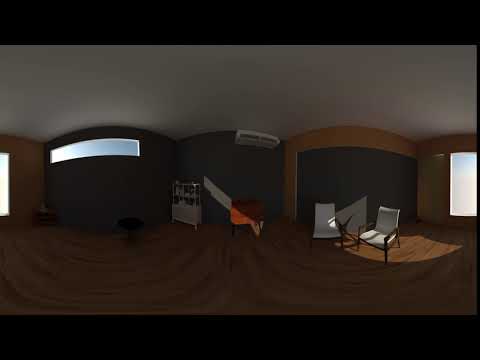The image appears to be a highly detailed, digitally-manipulated photograph of an indoor living space, possibly generated by AI. The room features a brown hardwood floor that occupies the bottom third of the image, leading to a variety of furniture and architectural details. Prominently positioned in the middle is a reddish-orange chair, above which hangs a white ceiling-mounted air conditioning unit. To the right of this chair are two white armchairs with black armrests. On the left, there is a bar cart and a wall with a large white window. 

The intricate image also displays several windows; a narrow vertical window on the far right wall, a half-window on the left brown wall, and another long, narrow rectangular window on a grey wall showing a blue sky. The background includes a mix of brown and grey walls, with a part of the right wall possibly featuring grey sliding doors or curtains. The ceiling is white and comprises the top third of the image.

The photograph is framed by a black header and footer, creating a distinct boundary for the detailed scene within. The artistic manipulation of the image uses a curvature effect, making the wooden floor slats and the walls bend outward and giving the impression that the image could form a continuous cylindrical panorama if wrapped around. Overall, this unique living room setup exudes a modern, relaxed atmosphere, highlighted by varied textures and colors.